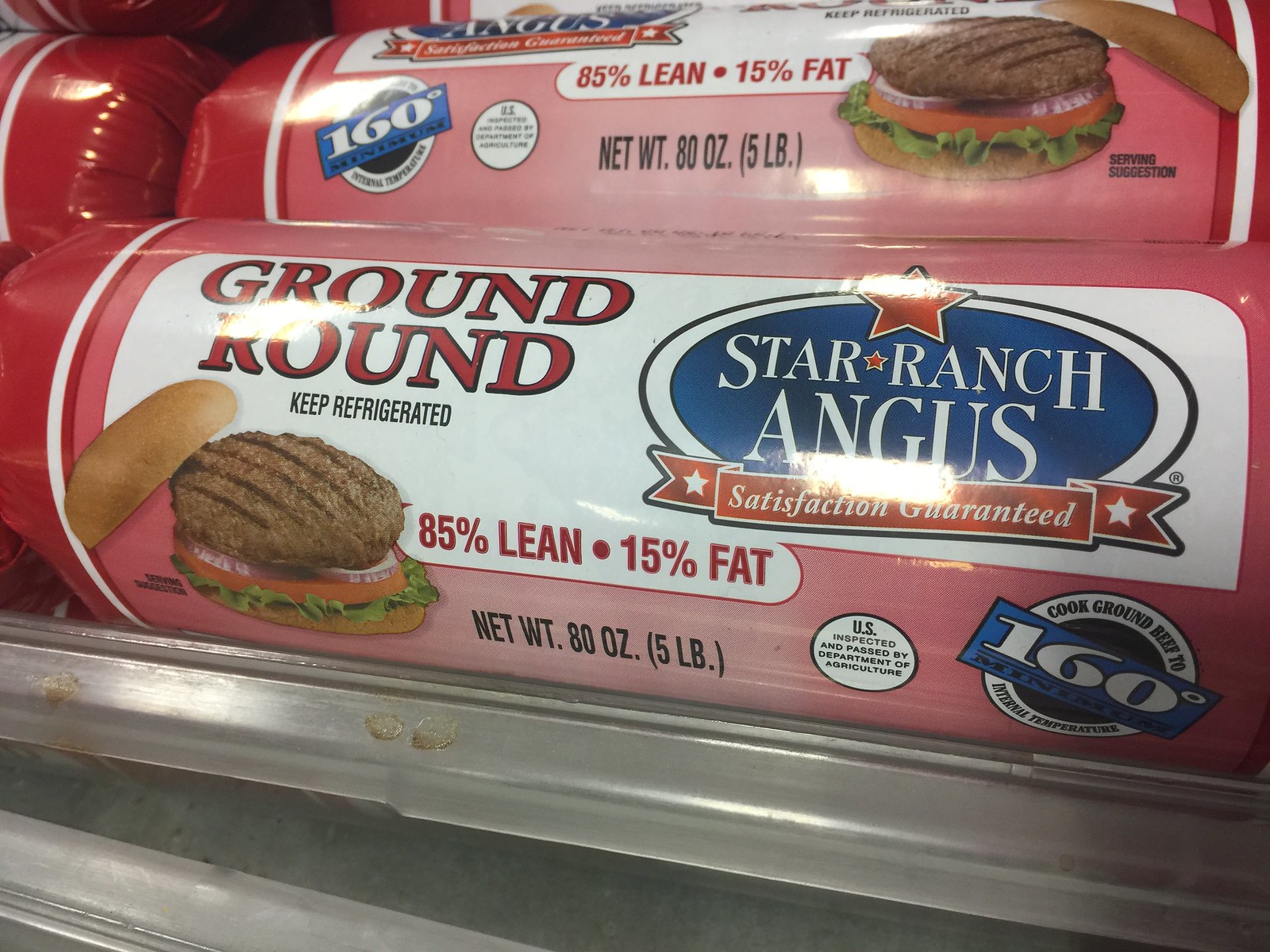Detailed Caption:

This close-up image showcases a package of Angus beef, prominently focused on two large portions situated in the center, with two partial portions visible on the left-hand side and a small sliver of a fifth portion in the background. The packaging features a distinct label with dark red outer edges and a thin white bordering line, set against a predominantly pink background. At the top, bold red text displays "Ground Round," with smaller black text beneath it stating "Keep Refrigerated." An appetizing image of a burger with lettuce, tomato, and onion beneath the patty graces the label. The burger’s bun is depicted slightly separated, with the bottom bun in place.

The packaging provides key nutritional information in red text, indicating "85% Lean, 15% Fat" and specifies the net weight as "80 ounces." Additionally, it gives a cooking guideline, advising to cook the ground beef to an internal temperature of 160 degrees Fahrenheit. Prominently, the brand name "Star Ranch Angus" is displayed in white text over a blue circular background, encircled by a white ring with a red star. Below the brand name, the packaging assures "Satisfaction Guaranteed" against a red backdrop, emphasizing the brand's commitment to quality.